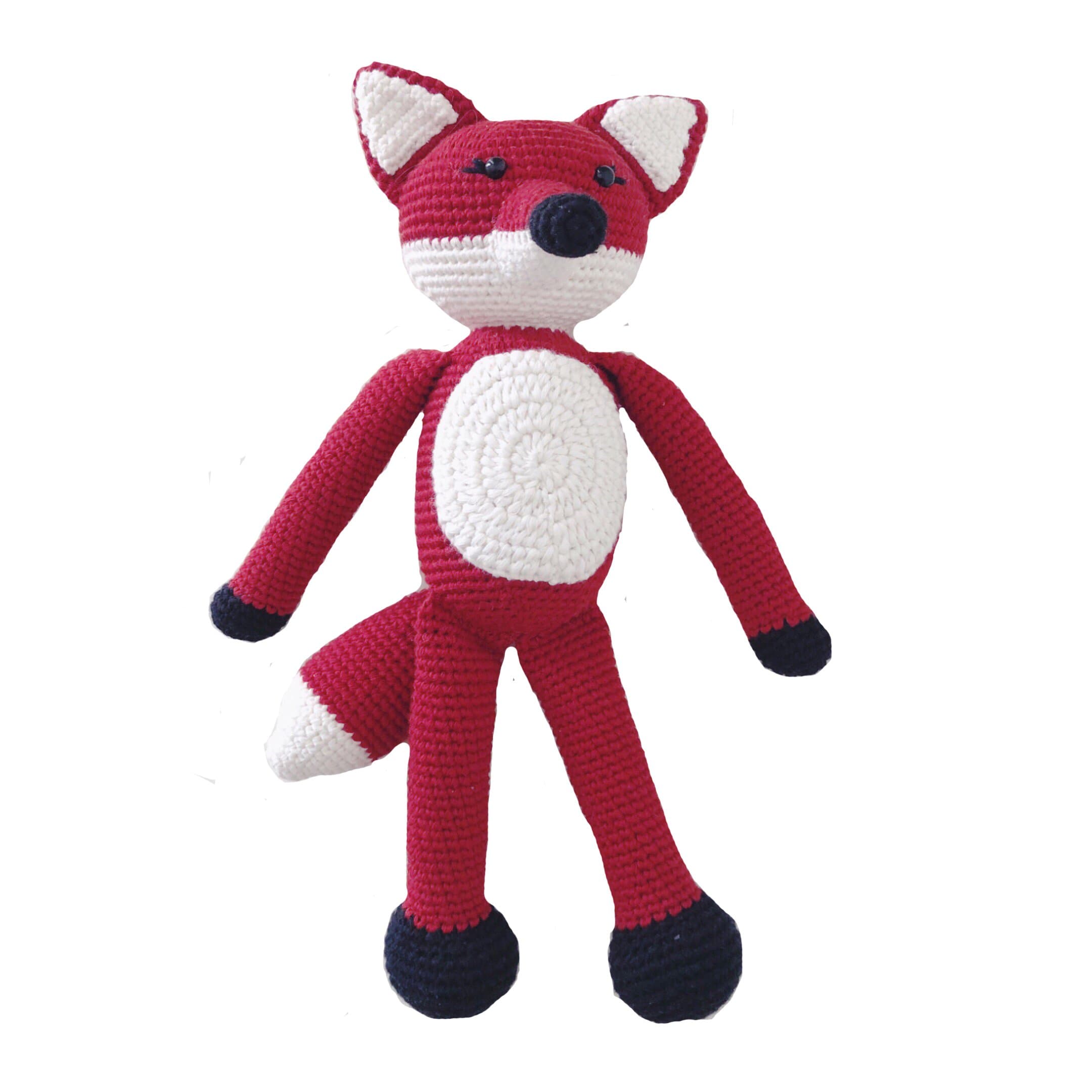The image is a detailed close-up of a handmade Amigurumi red fox, crafted with evident care. The fox, distinctly characterized by its vibrant red body, features black rounded paws and feet. Displaying traditional Amigurumi styling, it has prominent white sections on its tail tip, belly, and lower face. The belly showcases a beautifully crocheted white magic circle pattern with multiple layers, adding depth to its texture. Its expressive face includes two black beady eyes and a black nose, with the nose tip contrasting against the red snout. The ears are predominantly red with white inner details. The fox is stuffed and stitched together, suggesting it was made by hand, possibly designed as a children's toy. Captured on a white background, the photo is taken from an overhead angle, emphasizing the detailed craftsmanship and soft texture of the toy.